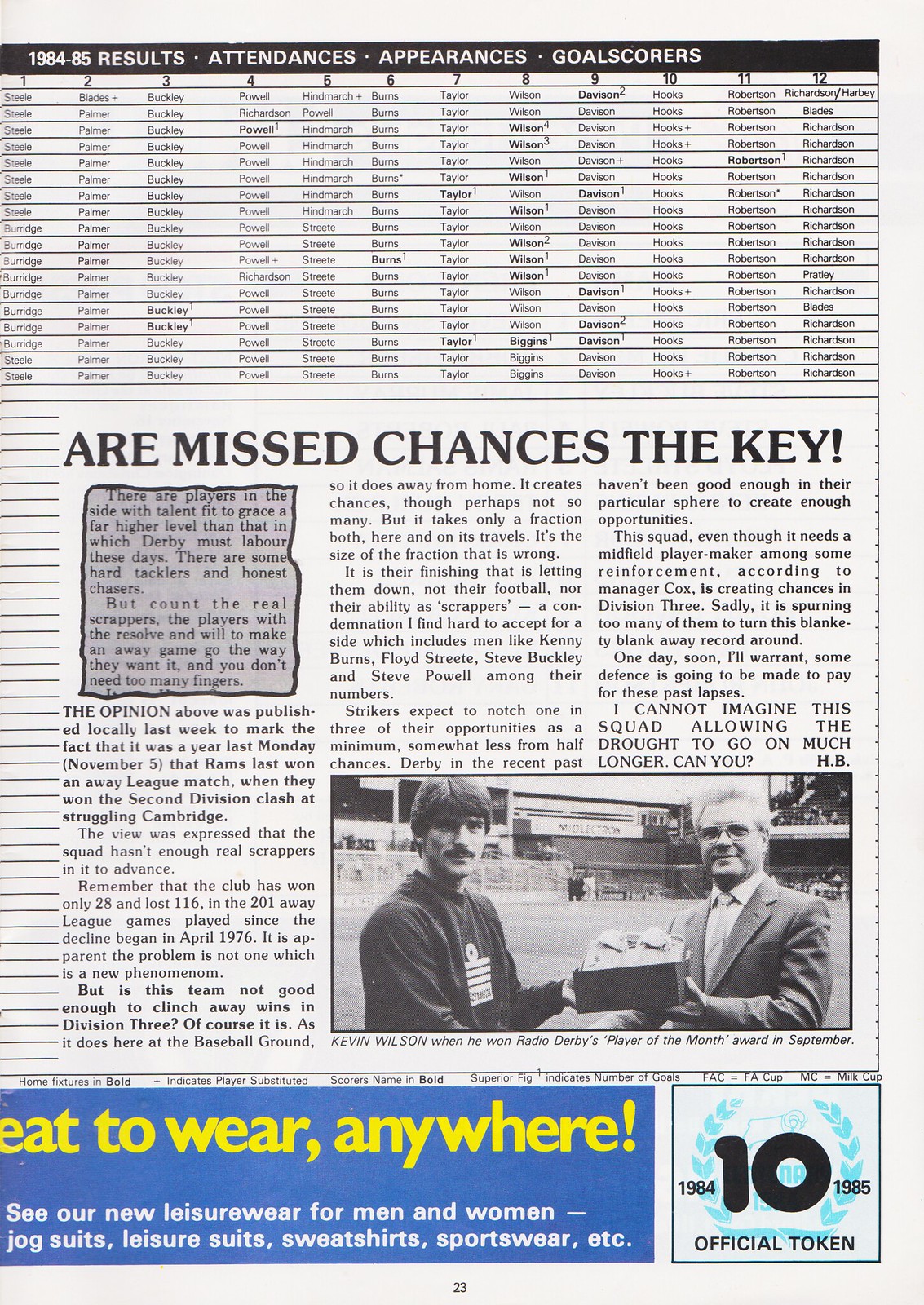This image captures a black and white page from a sports magazine, prominently featuring an article and an award presentation. At the top, a black horizontal bar displays the title "1984-85 results, attendance, appearances, and goal scores," followed by columns and rows of names beneath it. Below this section, there's an article titled "Are Missed Chances the Key?" with the first two paragraphs outlined in black felt pen. Towards the middle bottom right of the page, a black and white photograph depicts two men, one with dark hair and the other with gray hair, holding a box-like award together in front of some buildings. The photo is labeled "Kevin Wilson when he won Radio Derby's Player of the Month Award in September." Additionally, the page includes an advertisement with a blue background and yellow text, as well as smaller banners with partially legible captions such as "eat to wear anywhere" and "10 in the box official token."